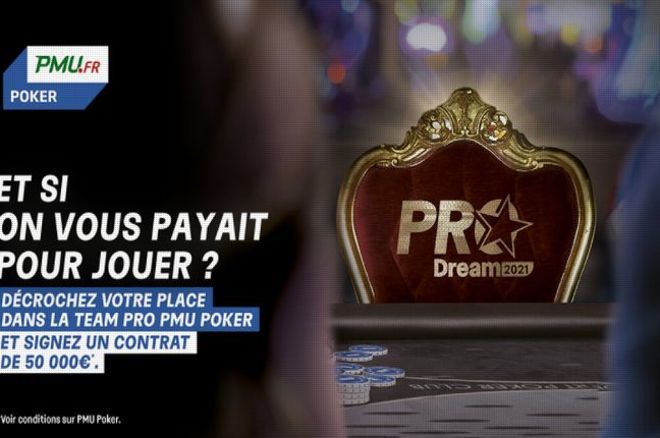The image depicts a sophisticated advertisement for a French poker game, primarily showcasing a luxurious chair with a red satin backing and a gold frame, emblazoned with "Pro Dream 2021" in gold lettering. The chair is positioned next to a gray poker table scattered with blue chips. On the left side of the image, white French text promotes the poker game, mentioning a contract worth 50,000 euros. An official-looking logo at the top left corner reads "PMU.FR," with the word "POKER" prominently displayed in a blue box beneath it. The scene is framed by the blurred outlines of people standing nearby, one in blue and another in red, adding depth to the image. The photograph combines realistic elements with sharp graphic design, creating a visually striking and detailed composition.